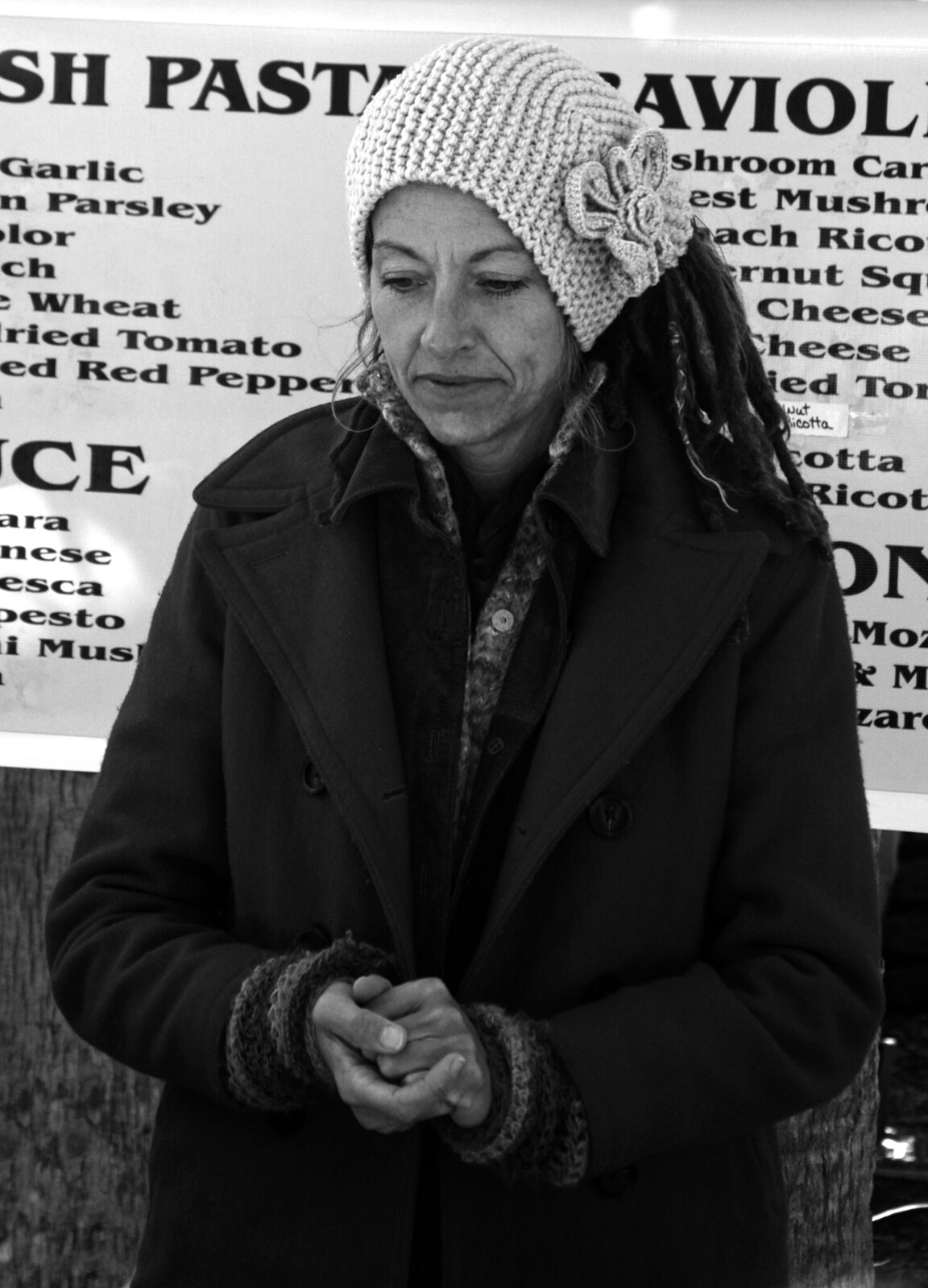This black and white photograph captures a middle-aged white woman standing outdoors in front of a sign listing various food items. She wears a knit cap adorned with a flower on the side, and her long dreadlocks can be seen at the back of her head. The woman’s attire suggests cold weather; she is dressed in multiple layers, including a heavy overcoat with bands on the collar and sleeve hems, a visible buttoned shirt, and possibly a sweater underneath. Her hands are clasped together in front of her as she looks slightly downward, giving an impression of contemplation or modesty. The sign behind her, partially obscured by her head, appears to offer an assortment of foods such as mushrooms, butternut squash, cheese, garlic, parsley, wheat, tomato, red pepper, and possibly pesto. A dark wall is also faintly visible behind her. The detailed layers of clothing and the list of foods in the background suggest she could be involved in a community or nonprofit activity, such as working at or visiting a soup kitchen.